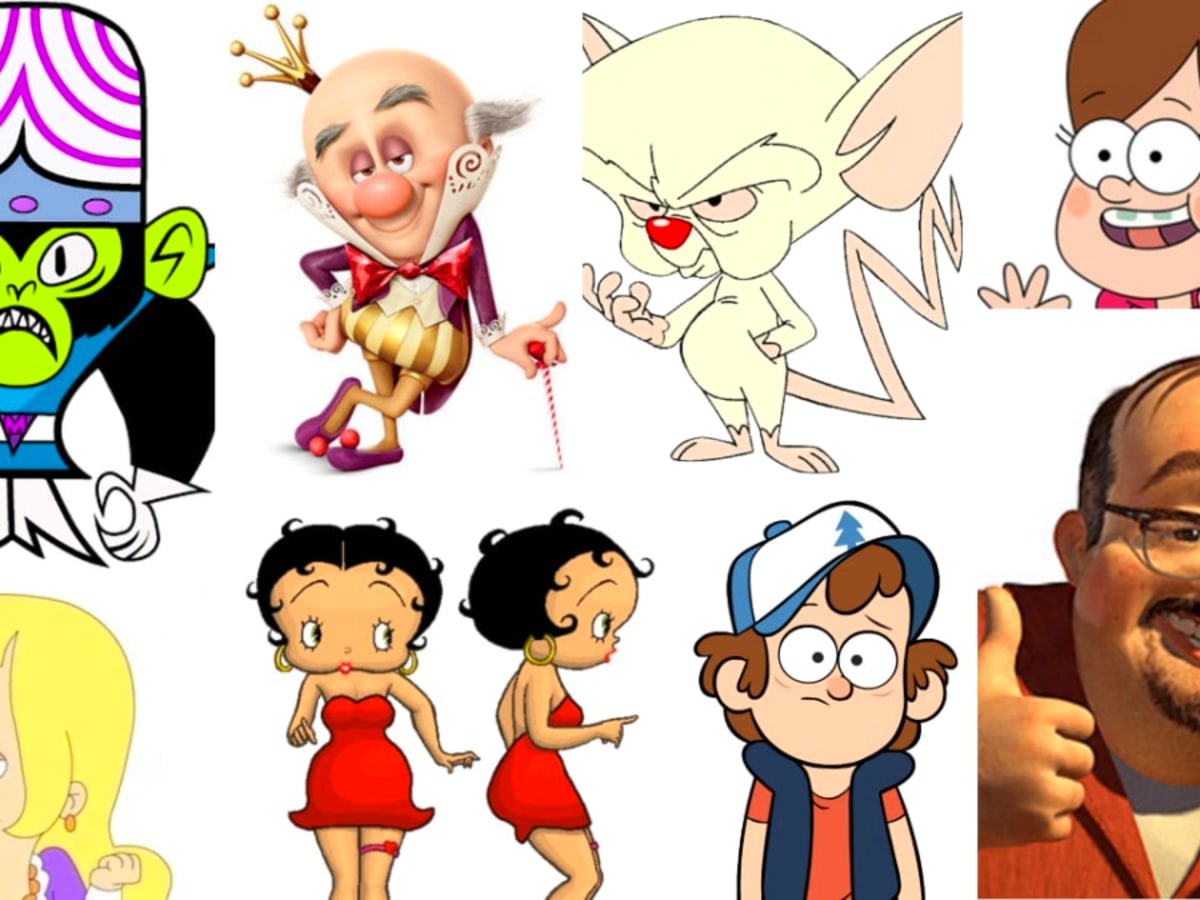The image features an array of nine detailed cartoon character decals displayed across two rows, with the top row comprising four characters and the bottom row featuring five. Starting from the top left, there's Mojo Jojo from the Powerpuff Girls, recognizable by his green face, black fur, white and purple helmet, and visibly angry expression. To his right, the Candy King from Wreck-It Ralph boasts a golden crown, red bow tie, purple boots, and candy cane in hand, complete with a delighted smile. Next, Brain from Pinky and the Brain, identified by his red nose, pink tail, and large ears. The fourth character in the top row is a young girl with brown hair, suggested to be from a Cartoon Network show.

The bottom row begins with what appears to be a partially visible blonde-haired character, identified by an ear with an earring, followed by the iconic Betty Boop depicted twice in her classic red dress, showcasing different angles. Moving right, there's a character with a mixed skin tone and black hair, likely from the same Cartoon Network show as the girl above. Next is a boy wearing a blue and white cap, and finally, partially visible towards the right edge, is the collector, Al McWhiggin, from Toy Story 2, recognizable even though he is somewhat cut off.

This detailed lineup effectively captures the distinct and vividly colored charm of each character, bringing a sense of nostalgia and animation history.